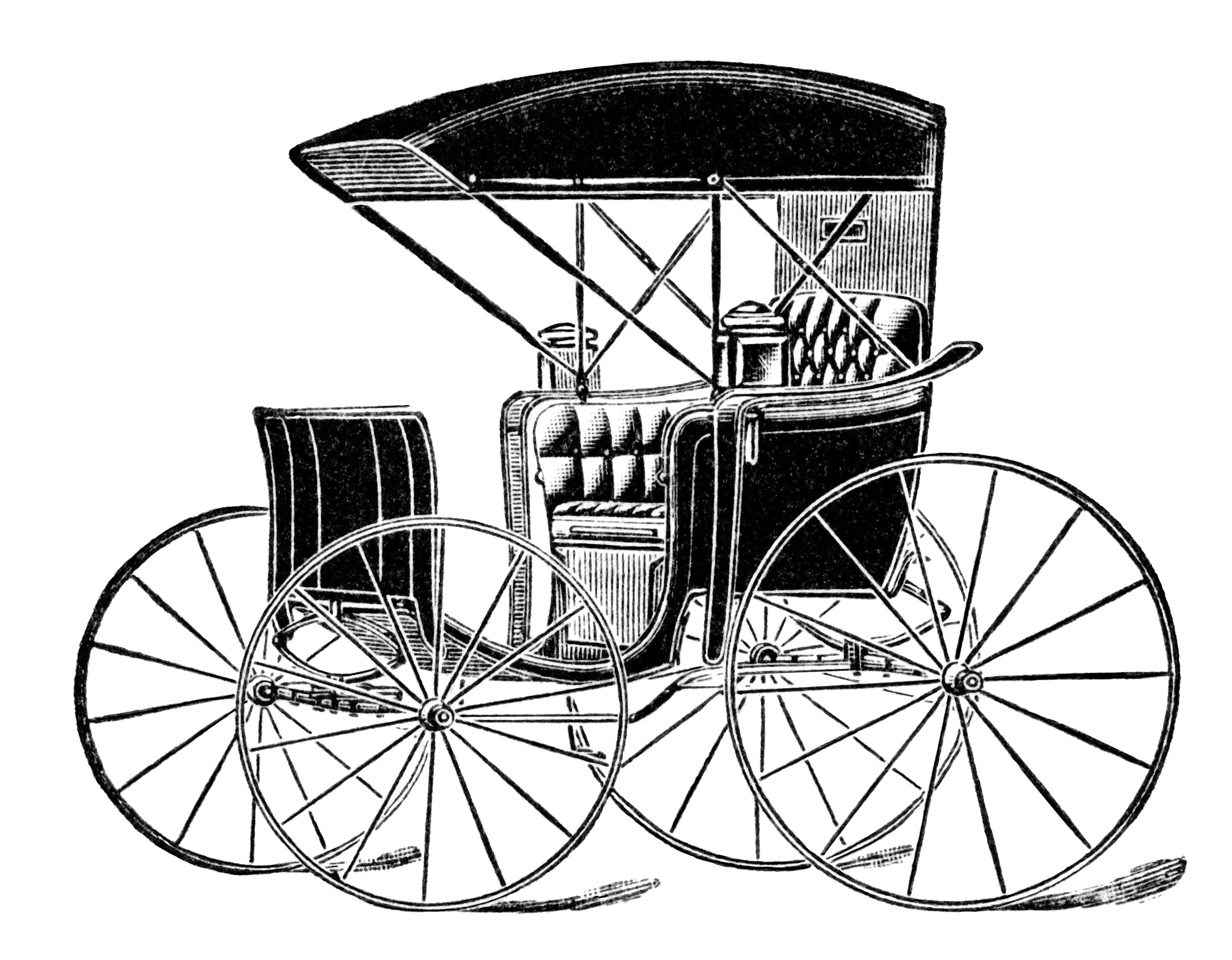The illustration depicts a horse-drawn carriage from an earlier era, meticulously detailed in black and white. The carriage features four prominent wheels, with the back wheels noticeably larger than the front. A cushioned two-seater bench is visible, suggesting a design meant for a well-dressed individual, perhaps in a suit or a fancy dress. The carriage has a black roof, providing partial cover while leaving the sides open to the air. There are two lights mounted on either side of the carriage, adding to its vintage charm. Additional details include a black climbing panel at the front and some noticeable marks near the wheels, enhancing the authenticity of the illustration. The smooth lines and careful craftsmanship make it a clear and recognizable depiction of a classic horse-drawn vehicle.